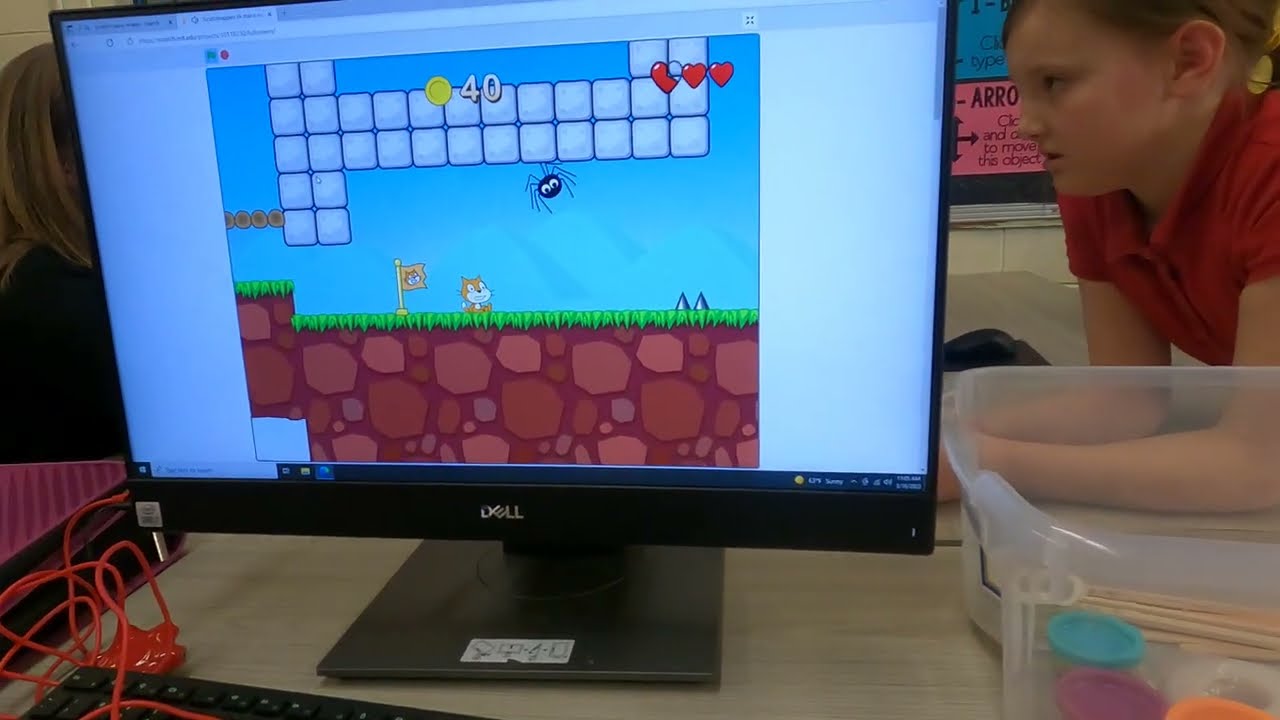The image depicts a school classroom scene with a Dell computer monitor prominently displaying a browser-based, old-school, 2D video game reminiscent of Super Mario Brothers. The game features a cartoon-like cat character running across a grassy area, with ice blocks suspended above and a dangling spider. The game interface shows three red hearts, a yellow circle with '40' next to it, indicating possibly coins, and various elements like brown earth and some grass. The monitor is placed on a light brown table. To the right of the monitor, a young blonde girl in a short-sleeved red polo shirt with a collar is looking intently past the screen, possibly at another person with shoulder-length blonde hair and wearing a black shirt, who is partially visible. Also present on the table are Tupperware containers, small canisters of Play-Doh, and blue, purple, and orange poker chips. Red cords are scattered around, hinting at a possibly interactive or educational setting. The background reveals instructional materials on a chalkboard, suggesting the game might be part of an early coding or educational activity.